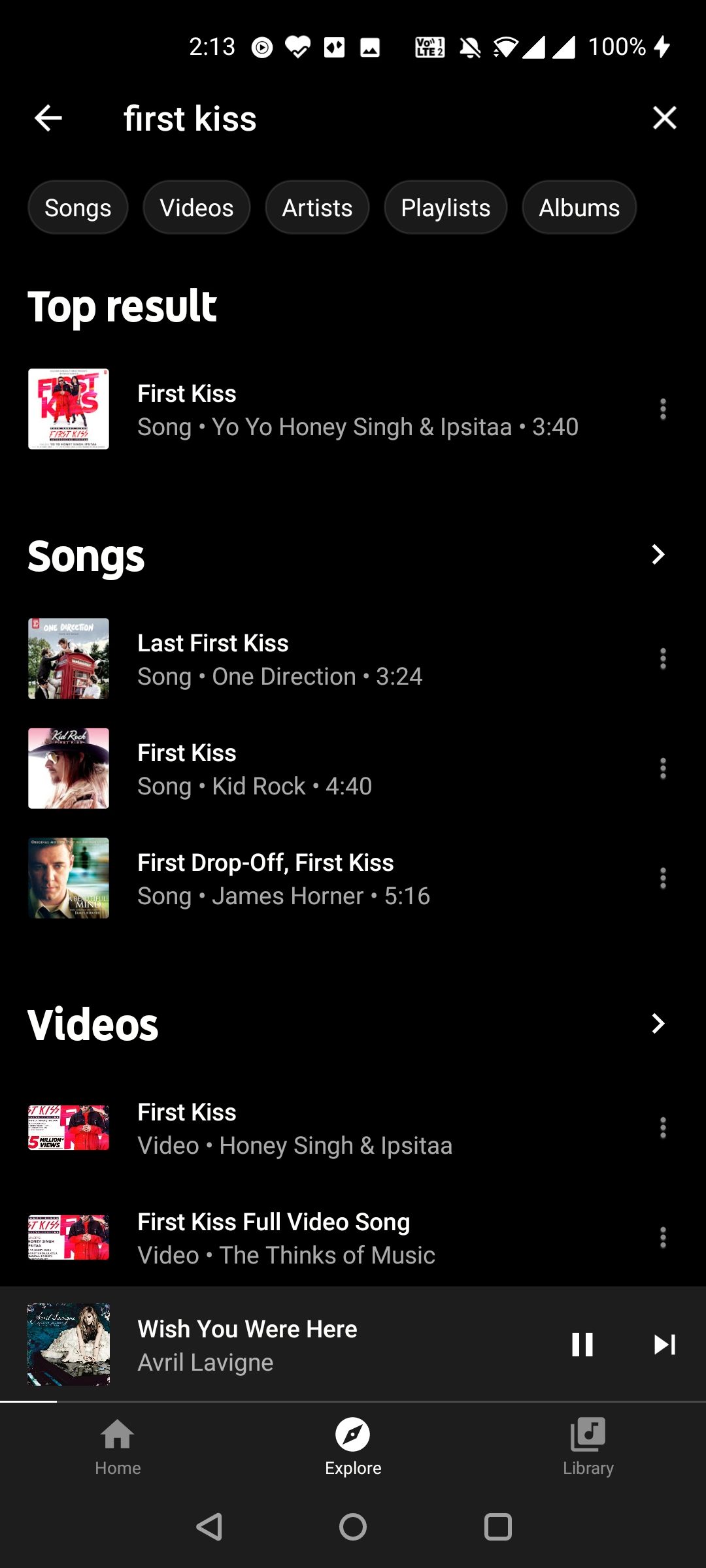The image is a screenshot of a smartphone display showing a media application interface. The background of the interface is predominantly black with a gray bottom section. The screen is currently in a section resembling a playlist or search result for audio content, such as a podcast or MP3 songs. At the very top of the screen, the text "First Kiss" is prominently displayed, indicating a search query or playlist name.

Below the title, the section labeled "Top Result" lists "First Kiss Song" as the primary result. Following this, there are categories labeled "Songs" and "Videos." Under the "Songs" category, three entries are listed, though the specific song titles are not detailed in this caption. Similarly, under the "Videos" category, three entries are shown, with the third video highlighted— "Wish You Were Here" by Avril Lavigne.

At the bottom of the screen, standard navigation buttons are visible: "Home," "Explore," and "Library." Additionally, the top banner of the interface is segmented into five tabs: "Songs," "Videos," "Artists," "Playlists," and "Albums." In the upper right-hand corner, a white "X" button is present for closing the current view. To the left-hand corner, a back arrow button is available for returning to the previous screen.